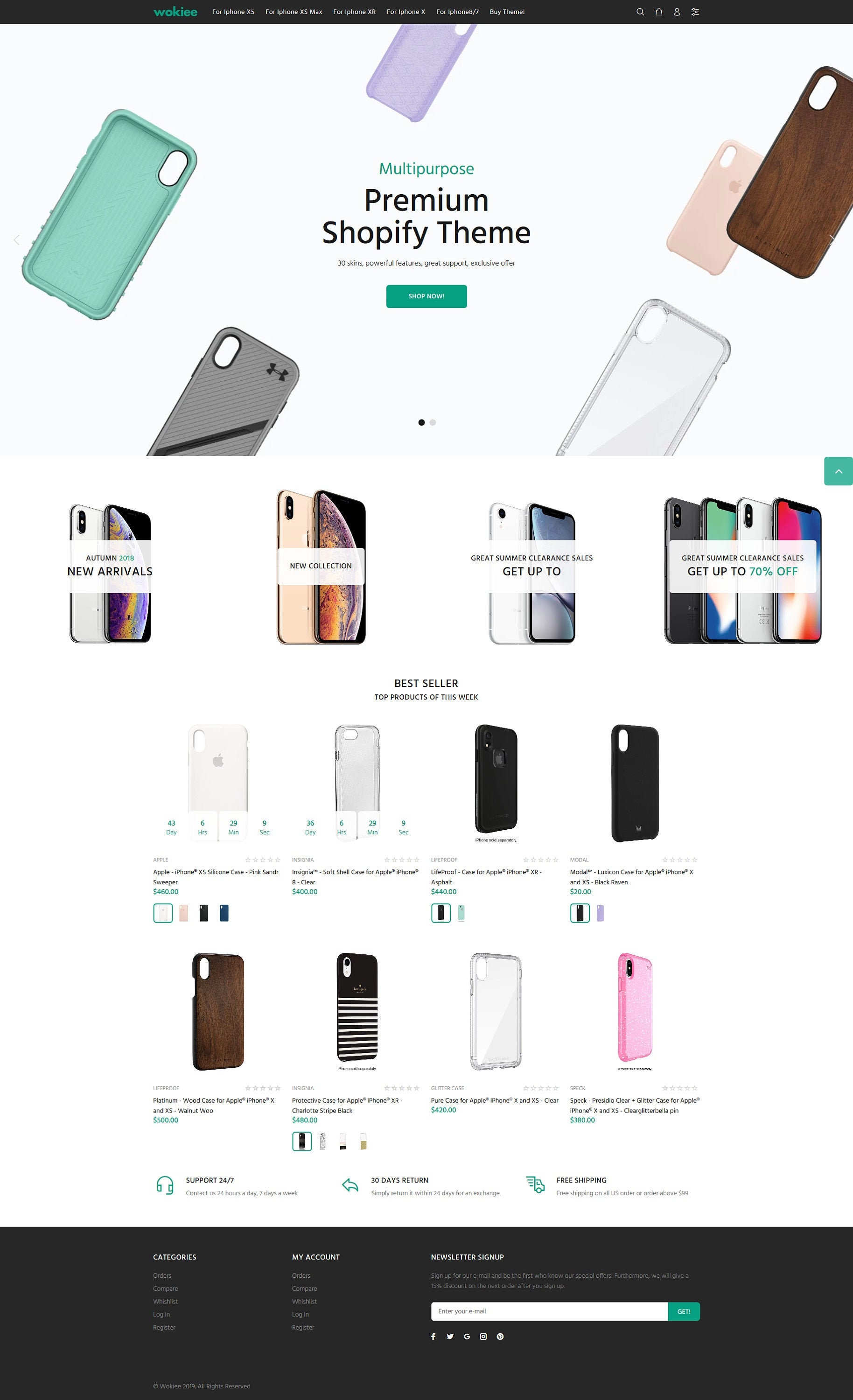The image contains a detailed layout featuring several key elements designed for a multi-purpose premium Shopify theme. 

At the top, there is a black rectangle with text. The word in green is unreadable, followed by additional text in grey, and small, unidentifiable grey symbols to the right.

Below, there's a display of various phone protectors in a range of colors: green, purple, grey with a black stripe, white, salmon, and brown. The title "Multi-Purpose Premium Shopify Theme" is prominently displayed, accompanied by smaller text that is unreadable. 

A green rectangle with unreadable text is also present. The image showcases numerous mobile devices categorized under different sections. Some callouts include "New Arrivals" and other unreadable headings. 

There are four phones below, segmented by messages such as "Get up to" and "70% off," although specific details are too small to discern. The "Bestseller" section highlights four different cases: two in white and two in black, with unreadable green and black text beneath each row.

Several green-outlined squares show various color schemes, including combinations of white, black, pink, and grey. Further down, another series of green-outlined squares are displayed, containing colors like black and possibly green or purple. This is followed by more images of phone counterparts in brown, black and white, white, and pink, again with small, unreadable text beneath them, primarily in black with some green text at the end.

Additional graphical elements include a headset icon in green with black text beside it, a right-facing arrow in green with adjacent black text that is too small to read, and other indistinguishable green symbols.

Towards the bottom, there is a black rectangle filled with white text, housing a smaller white rectangle with more writing and a green rectangle featuring two dots. Below this, a series of small symbols are present but are not identifiable.

Overall, the image is densely populated with colorful phone protectors, promotional text, and various symbols indicating a highly detailed template designed for an e-commerce Shopify theme.